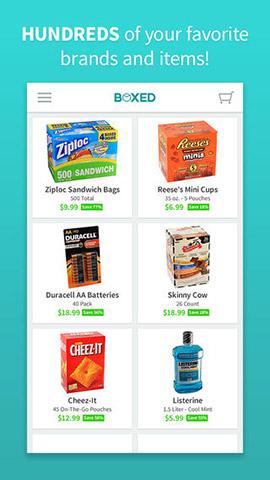In this screenshot, we observe a vibrant turquoise blue background. Centrally positioned is a large white rectangle, with dimensions resembling those of a phone or tablet screen, being taller than it is wide. 

At the very top, just above the white rectangle, there's a phrase in white letters reading "Hundreds of your favorite brands and items." Within the white rectangle, the layout is as follows:

The uppermost section features a narrow rectangle. On its left, there are three horizontal bars symbolizing a menu. Next to this, the word "Boxed" is written in turquoise. Towards the right side of this narrow rectangle, we see an icon of a shopping cart.

Below this, the main content is organized into three rows and two columns of displayed items, each available for addition to a shopping cart:
- **Top Left**: An image of Ziploc sandwich bags. Underneath the image, the title is in bold black letters with a smaller description in fine black print, and a price in green listed as $9.99.
- **Top Right**: A package of Reese's Mini Cups with a similar title and pricing format.
- **Middle Left**: Duracell AA batteries.
- **Middle Right**: A Skinny Cow product.
- **Bottom Left**: A box of Cheez-Its.
- **Bottom Right**: A blue bottle of Listerine.

Each product's price is prominently displayed beneath it, next to its description.